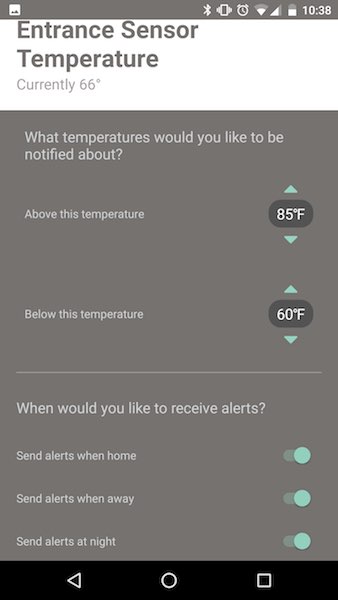This detailed screenshot from a mobile app displays the settings for an alarm system connected to an entrance sensor. At the top of the screen, a white background features a gray overlay text stating, "Entrance Sensor Temperature 66°F." Directly below, a section with a gray background and white text asks, "What temperature would you like to be notified about?" The user has selected to receive notifications if the temperature exceeds 85°F. Additionally, there is a command indicating a preference for maintaining the home's temperature at 60°F.

Further down, the user is configuring the notification settings for the entrance sensor by checking various options: notifications should be sent when the user is home, away (the second choice), and at night. This comprehensive setup suggests that the app enables users to monitor and manage the temperature via sensors throughout their home, ensuring they are alerted if the temperature rises above their desired threshold to maintain a consistent environment.